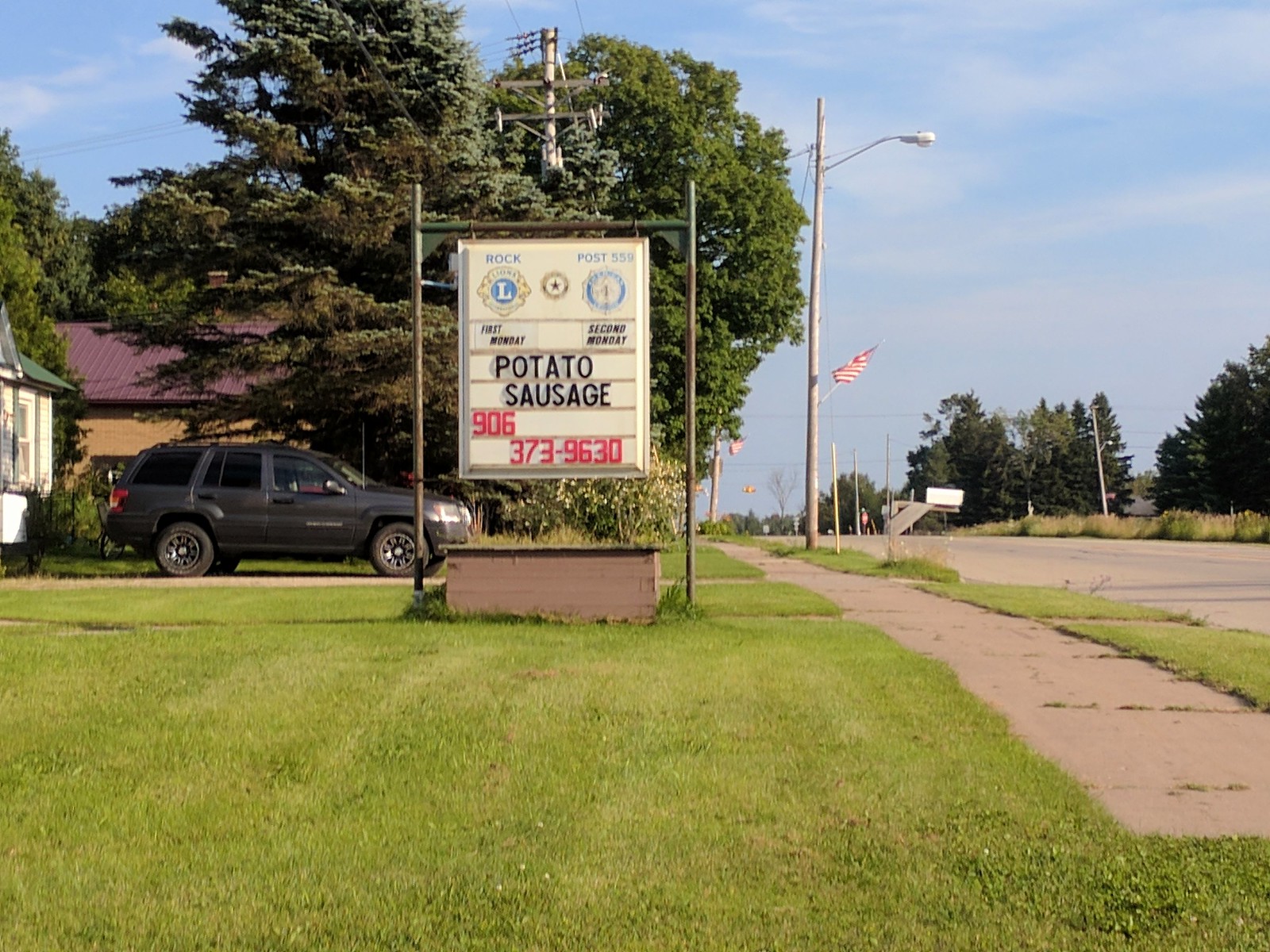In a peaceful Southern neighborhood with a clear blue sky, this photo captures the sidewalk in front of a well-maintained lawn adorned with several American flags. Prominently featured is a large sign from the Lions Club, characterized by its white background, gold trim, and blue ‘L’ logo, topped with a floral decoration and three circles. The sign advertises "Potato Sausage" in black text, followed by the contact number "906-373-9630" printed in red. Nearby, a dark gray Jeep Grand Cherokee is parked in the driveway. Surrounding the area, there are two houses; a white house just visible on the left and a brown house with a gray roof on the right. The scene is framed with big, bushy trees, light poles, and a mix of grassy patches and sidewalks, delivering a sense of serenity and community.